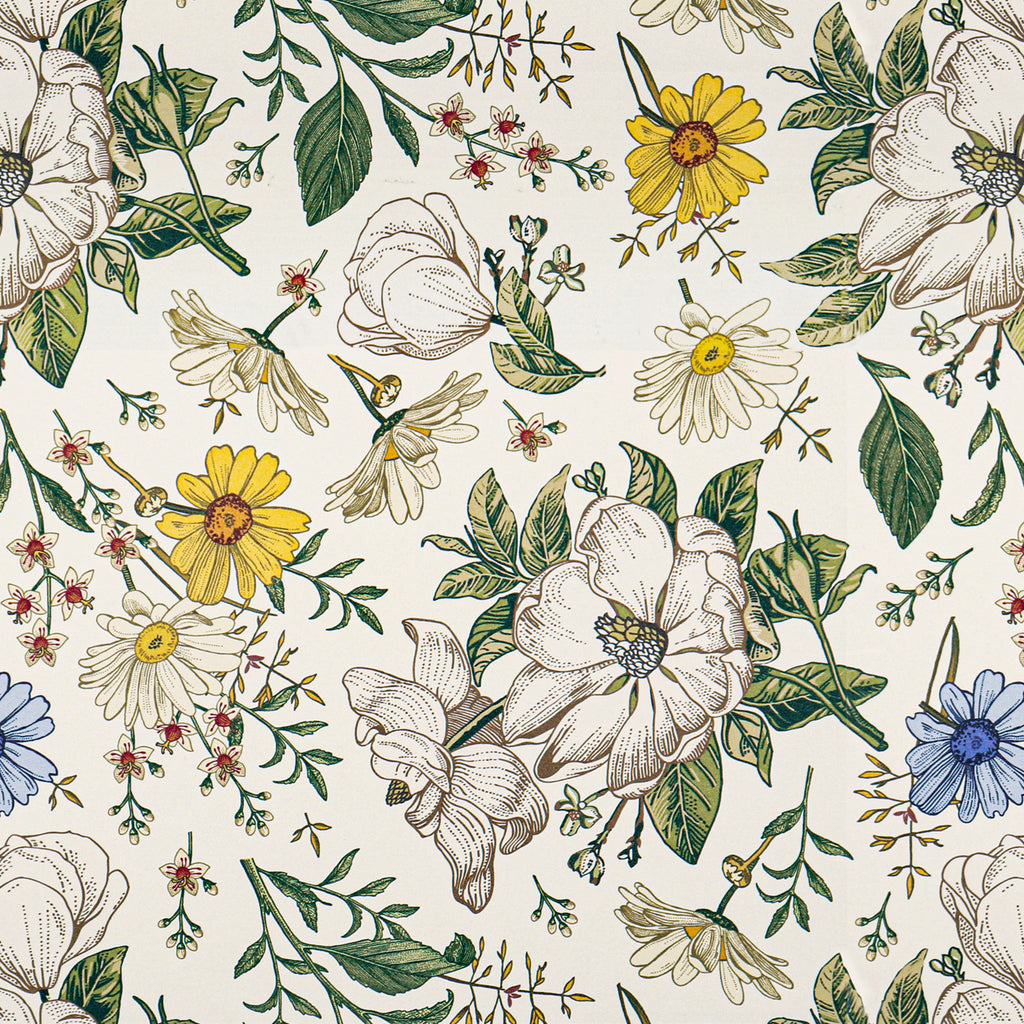The image depicts a square swatch of fabric or wallpaper showcasing a meticulously illustrated floral pattern. The repeat pattern features a variety of artistically drawn flowers, including daisies and larger blooms with white petals and conical-shaped centers, rendered in white, yellow, and light blue. Small accents of red highlight the centers of some smaller flowers. Intertwined with the flowers are green leaves and occasional short stems, enhancing the natural motif. The illustration employs line work and dot detailing for added texture and depth, set against an off-white background. The floral and foliage arrangement is rotational, contributing to a cohesive, repeating design that conveys an intricate yet stylized depiction of nature.